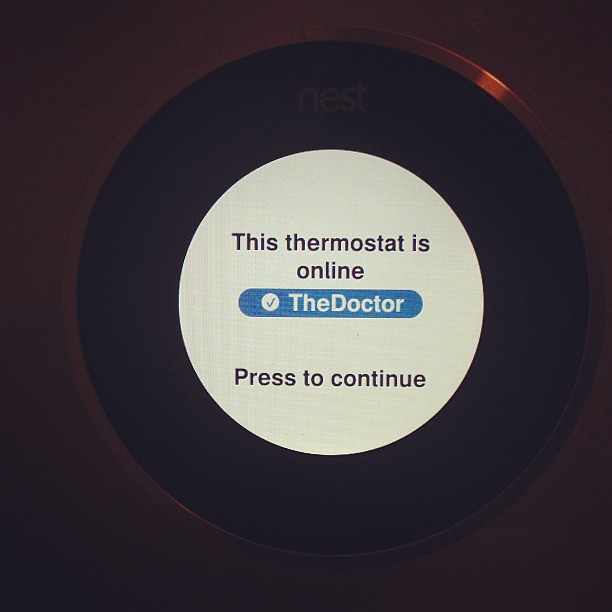The image features a slightly off-center, circular object positioned towards the right. The outermost part of this object is a metallic ring, colored in a shiny, reflective red with visible glare. Moving inward, there is a textured ridge followed by a black ring. At the top of the black ring, the word "Nest" is subtly imprinted in light text. 

At the core of the object, there is a white circle that contains the text "This thermostat is online." Within this white space, there is also an elongated blue oval featuring a check mark and the text "thedoctor" without any spaces between the words. Below this, in black text, it reads "Press to continue."

The background surrounding this central object, visible in the upper-left, upper-right, bottom-left, and bottom-right corners of the image, is a darker shade of red that harmonizes with the red of the metallic ring.